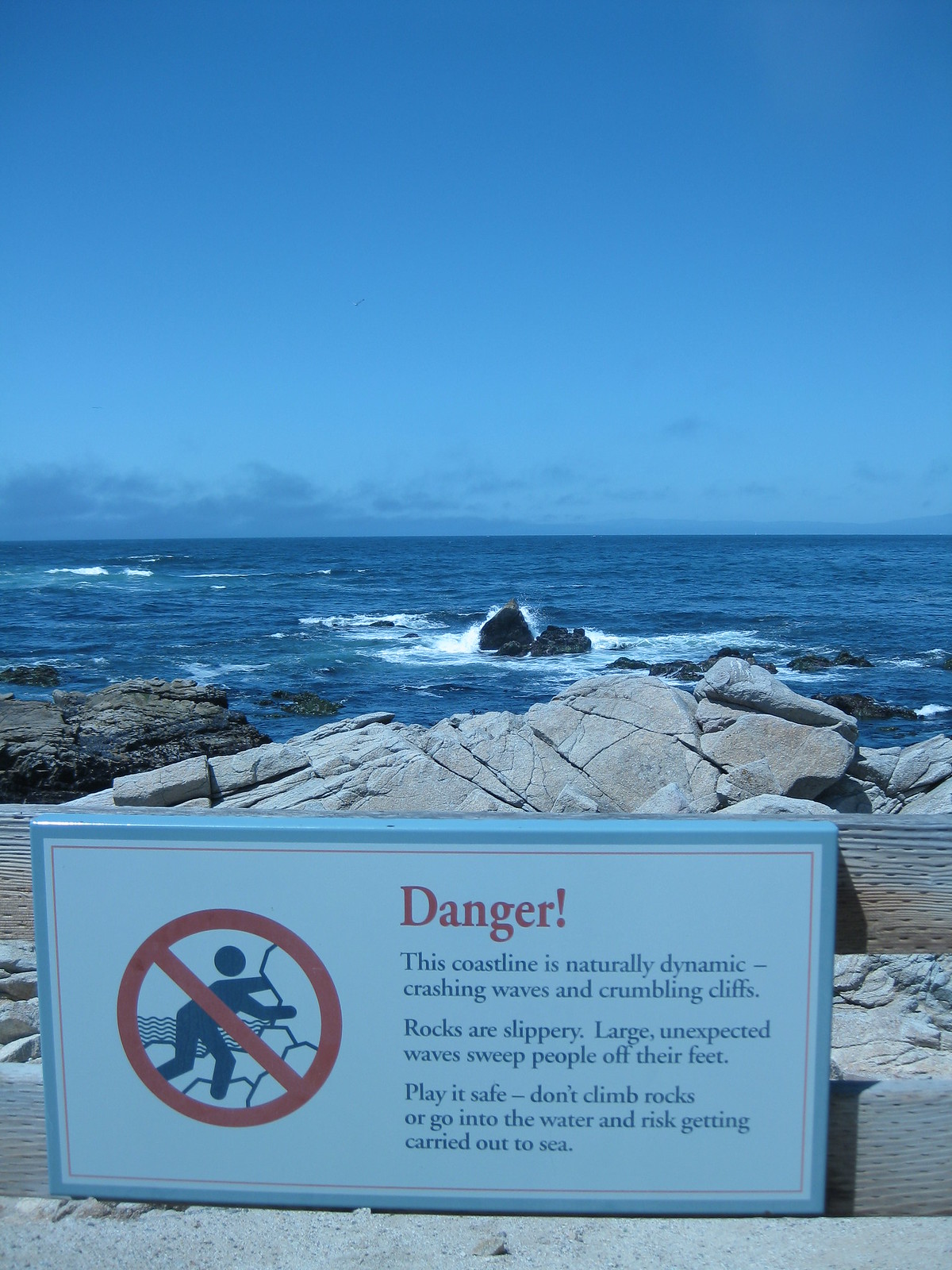The photograph captures a vivid, full-color scene of a rocky shoreline on a very clear day. The deep blue sky meets the equally blue water in the distance where a few wispy clouds float near the horizon. Jagged, dark gray and black rocks jut out of the water closer to the shore, with white foam crashing against them. More leveled and lighter-colored rocky areas suggest where one could potentially walk. In the foreground, a large sign with a blue border and white background warns of the dangers ahead. The sign features a bold red circle with a cross through an image of a person climbing rocks. Bold text declares "Danger" and details the perilous nature of this coastline: the dynamic nature of the crashing waves, the treacherous, crumbling cliffs, and the slippery rocks. It continues to warn that large, unexpected waves can sweep people off their feet, urging onlookers to play it safe by avoiding climbing on the rocks or entering the water, as they risk being carried out to sea. Below this area, some sand is visible, suggesting the presence of a beach. The photo conveys both the beauty and the inherent dangers of this natural landscape.